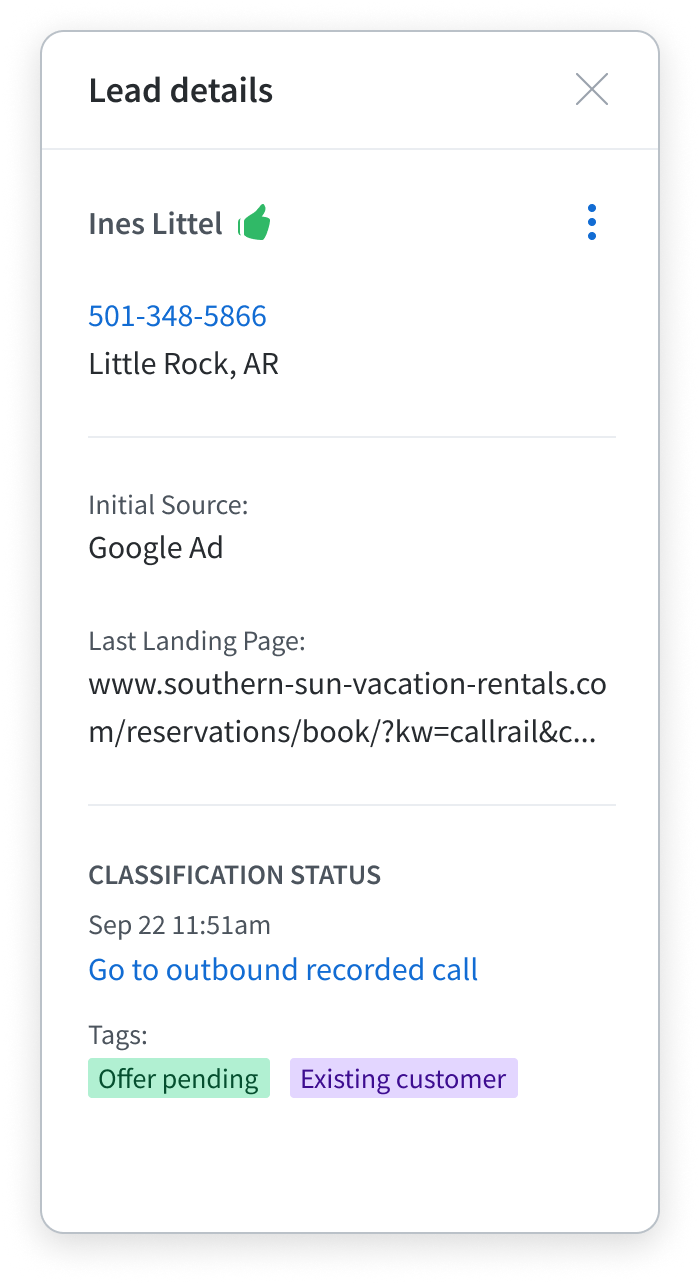A screenshot of a detailed pop-up window titled "Lead Details." The pop-up indicates that it has been approved by Ines Little, symbolized with a thumbs-up icon. The information includes a GPS coordinate labeled "5013485866" situated in Little Rock, AR. The lead source is identified as a Google advertisement. The last landing page visited is specified with a full URL to the Southern Sun vacation rental website. The lead was classified on September 22nd at 11:51 AM. There is a blue hyperlink labeled "Go To Outbound Recorded Call" for further action. Two tags are visible: "Offer Pending" in turquoise blue and "Existing Customer" in purple.